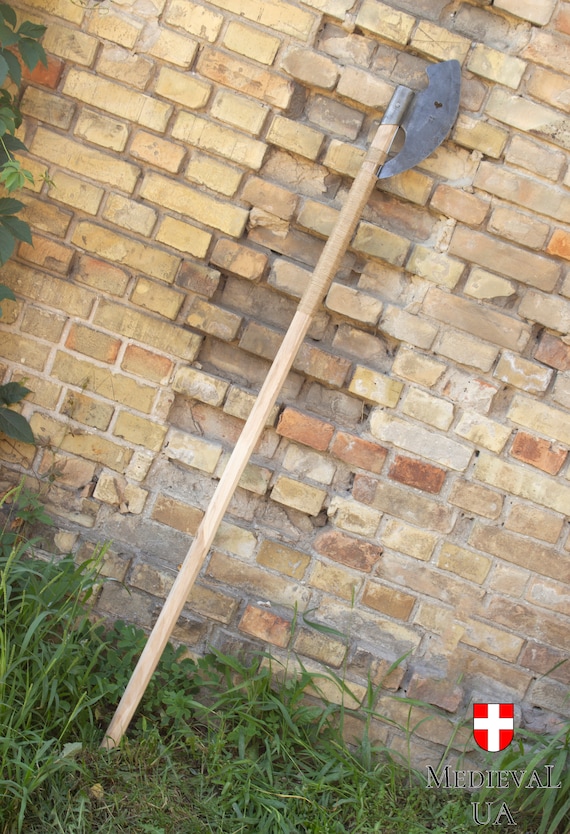The photograph depicts a medieval halberd, a long wooden weapon with a curved axe blade, leaning against a uniquely textured brick wall. The weapon's metal cap, featuring a heart-shaped cutout, rests on a patch of ankle-high grass and overgrown vegetation at the wall's base. The brick wall, made of varied-colored bricks ranging from tan to dark brown, appears repaired or reconstructed due to its mismatched mortar and bricks. The image, taken at a slight 30-degree tilt to the right, also includes a logo in the bottom right corner—a red shield with a white cross and the text "Medieval UA" beneath it. The overall scene is captured in a clear, realistic style, highlighting the distinct elements of the aged wall and historical weapon.